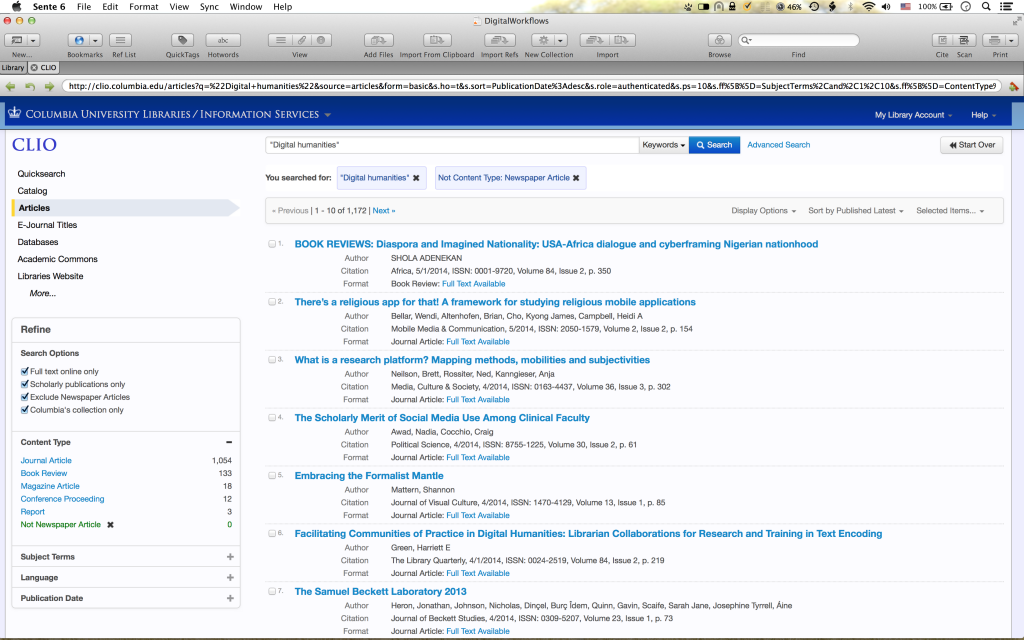**Detailed Caption:**

This is a detailed screenshot of a university library's webpage. At the very top, the computer's utility bar is visible, featuring a black Apple logo on the far left. To the right of the logo, bold black text reads "Cente6". Further right, there are grey menu options including "File", "Edit", "Format", "View", "Sync", "Window", and "Help". The top right corner is populated with numerous symbols: a grey bear paw print, a black and white bar, an arch shape, a black lock, a yellow circle with a black checkmark inside, a round black icon with "46%", a black circle with an arrow, a black scroll of paper, the Bluetooth logo, the Wi-Fi logo, a volume icon, the American flag, a battery symbol displaying "100%" with a plug icon in the center, a clock with a grey outline, a magnifying glass, and three lines with three dots.

Beneath this utility bar, the webpage itself has a predominantly white background. The content is organized into sections, each marked by a blue header. Under each blue header, three subsections are formatted with grey text labeled "Author", "Citation", and "Format".